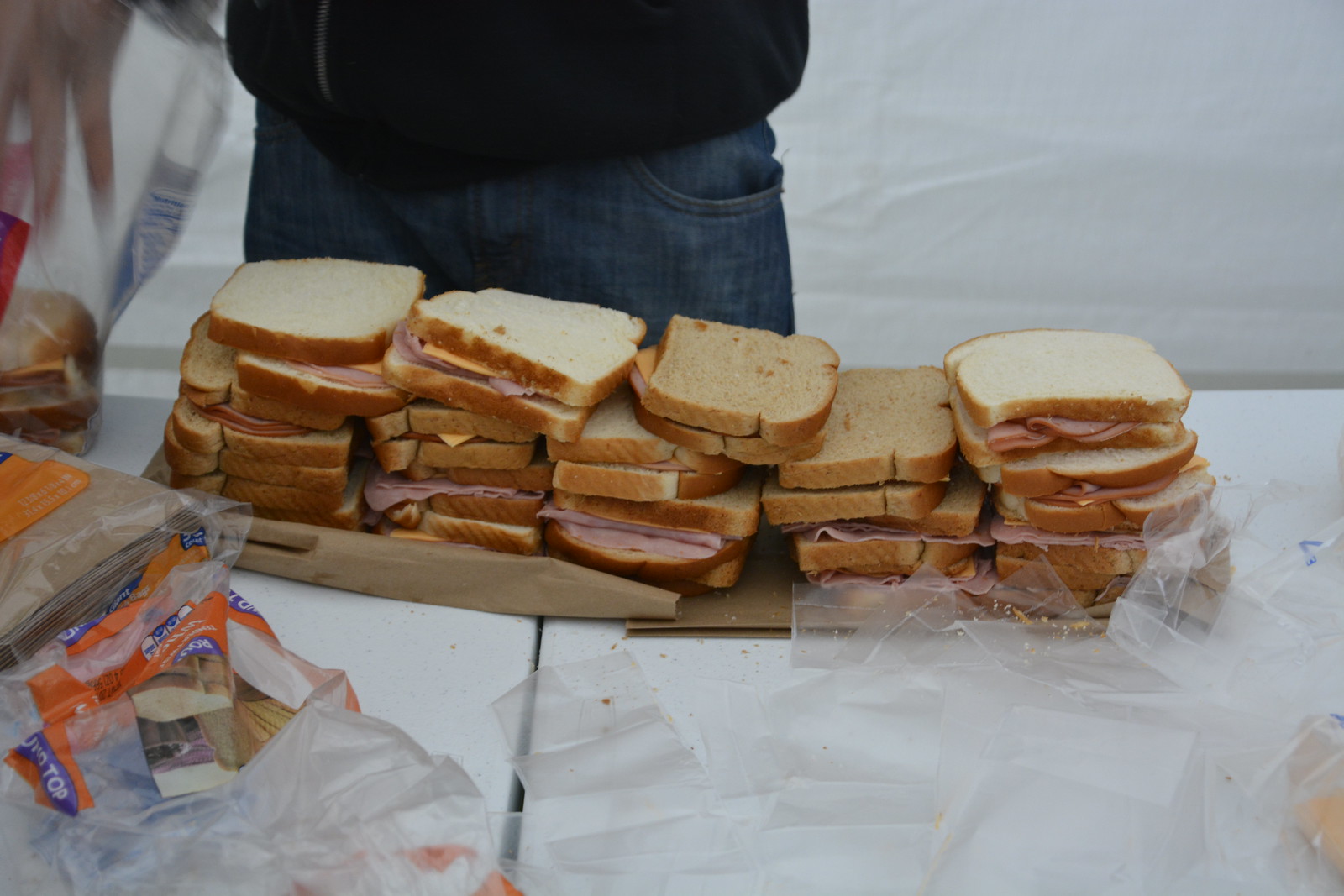The image depicts a large assortment of ham and cheese sandwiches stacked haphazardly on a white table covered with a brown cardboard sheet. The sandwiches, some made with white bread and others with wheat bread, are piled three to five layers high, forming an impressive heap. Slices of orange cheese and pink ham peek out from between the slices of bread. In front of the sandwiches are several plastic wrappers, likely from bread loaves, displaying orange and blue designs. To the side, there are additional loaves of bread and a plastic bag filled with brown paper bags, possibly for distribution. A person, dressed in blue jeans and a dark blue sweatshirt, stands behind the table, visible from mid-upper thigh to torso, suggesting a setting where food is being prepared or distributed, potentially for a charitable event like a homeless shelter.